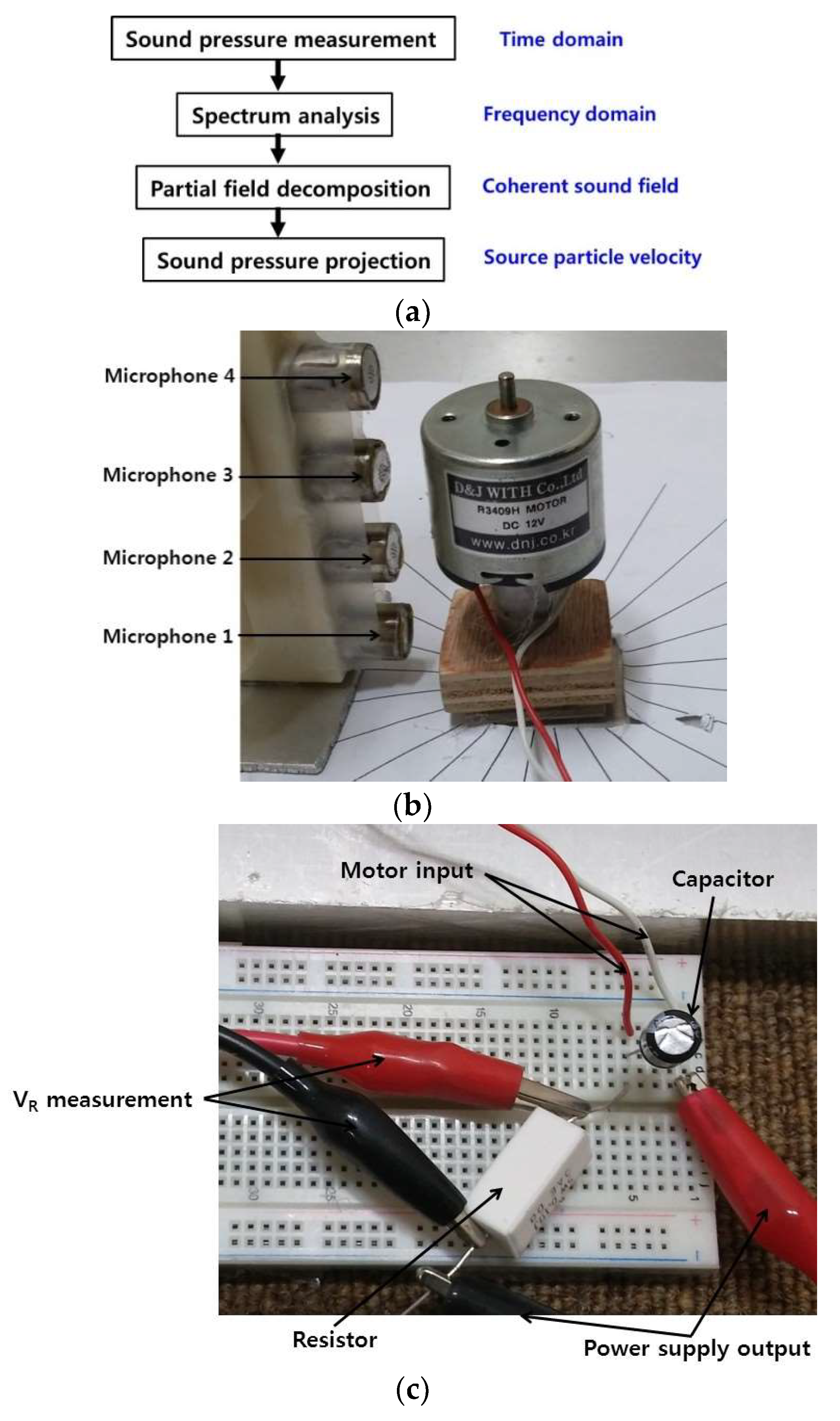The image is a comprehensive diagram featuring a flowchart and two detailed photographs, annotated with various labels. At the top of the image is a flowchart laid out with black text reading "sound pressure measurement," leading via downward arrows to "spectrum analysis," "partial field decomposition," and finally "sound pressure projection." On the left of the flowchart, blue text aligns with each stage: "time domain" corresponds to the first stage, "frequency domain" to the second, "coherent sound field" to the third, and "source particle velocity" to the fourth.

Below the flowchart is the first photograph (Figure B), showcasing a cylindrical metal device, identified as a DC motor labeled "D and J with Company Limited, R3409H motor, DC 12V," attached to a wooden base. The motor has red and white cables extending from it, consistent with the observed theme of red and white wiring throughout the image. To the right of the motor is a stack of small cylindrical devices, labeled "microphone 4" at the top and proceeding down through "microphone 3," "microphone 2," to "microphone 1," as indicated on the left side of the image.

The second photograph (Figure C), positioned at the bottom, depicts a white board filled with various electronic components. This includes a metal pin with red and white wires affixed to it, and a red clamp connected to the pin. Adjacent to the pin is a small white box, described as a power supply output, with a red clamp on one side and a black clamp on the other. The schematic labels this section extensively with terms such as "VR measurement," "resistor," "motor input," and "capacitor," clearly pointing to the respective components connected by metal wires and clamps.

Overall, the caption provides a detailed representation of a sound pressure measurement and analysis setup, displaying both the theoretical flow from sound pressure measurement through to projection, and the practical components involved like the DC motor, microphones, and electronic circuitry essential for the process.